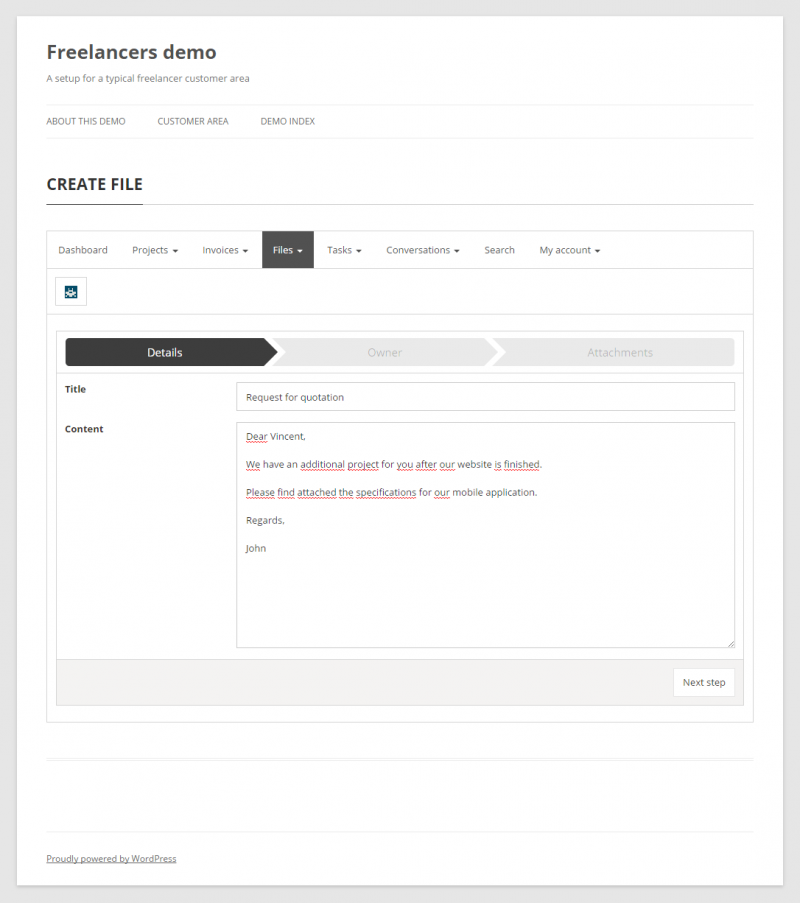This image is a detailed screenshot of a freelancer's demo interface designed for managing customer interactions and projects. The interface is titled "Freelancer's Demo: A Setup for a Typical Freelancer Customer Area." It features three main navigation tabs: "About This Demo," "Customer Area," and "Demo Index."

Below this header, a more elaborate navigation panel is present with tabs labeled "Create File," "Dashboard," "Projects," "Invoices," "Files," "Tasks," "Conversations," "Search," and "My Account." Each of these tabs, except "Dashboard" and "Search," has a small black arrow indicating dropdown options for further actions.

The current view is focused on the "Files" tab, with the "Details" subsection highlighted in black. Adjacent tabs labeled "Owner" and "Attachments" are shown in light gray, indicating subsequent steps. In the "Details" section, there are input fields for "Title" and "Content." The "Title" field is filled with "Request for Quotation," and the "Content" field displays a message from a client: 

"Dear Vincent,  
We have an additional project for you after our website is finished. Please find attached the specifications for our mobile application.  
Regards, John."

At the bottom right corner, a "Next Step" button is visible, which presumably will guide the user to the "Owner" and then the "Attachments" sections, completing the process for creating and sending the file.